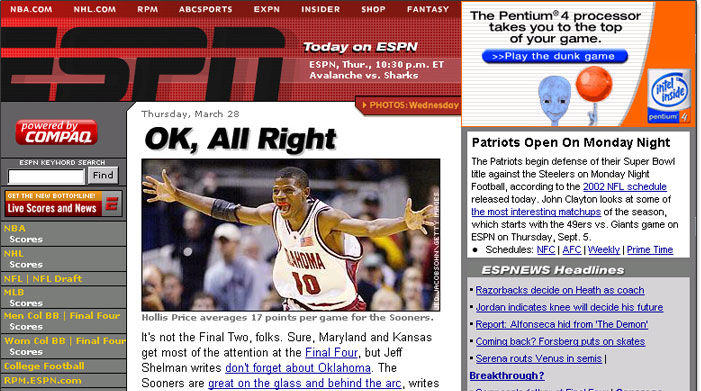In this detailed image of an ESPN webpage, several categories are prominently displayed, including NBA.com, NHL.com, European Sports, ABC Sports, EXPN, Insider, Shop, and Fantasy. The focal point of the webpage highlights the ESPN Thursday schedule with a notable game between the Avalanche and the Sharks set for 10:30 PM Eastern Time on Thursday, March 28th. A featured article spotlights the performance of a player from the Sooners, noting an average of 17 points per game. Additionally, the coverage includes insight from Jeff Shulman, who urges readers not to overlook Oklahoma amidst the Final Four excitement, which is typically dominated by teams like Maryland and Kansas. The article praises the Sooners' strong rebounding and three-point shooting abilities. The webpage is powered by Compaq and promotes live score updates and news through its "bottom line" feature. For further details and information, viewers are directed to visit ESPN.org.